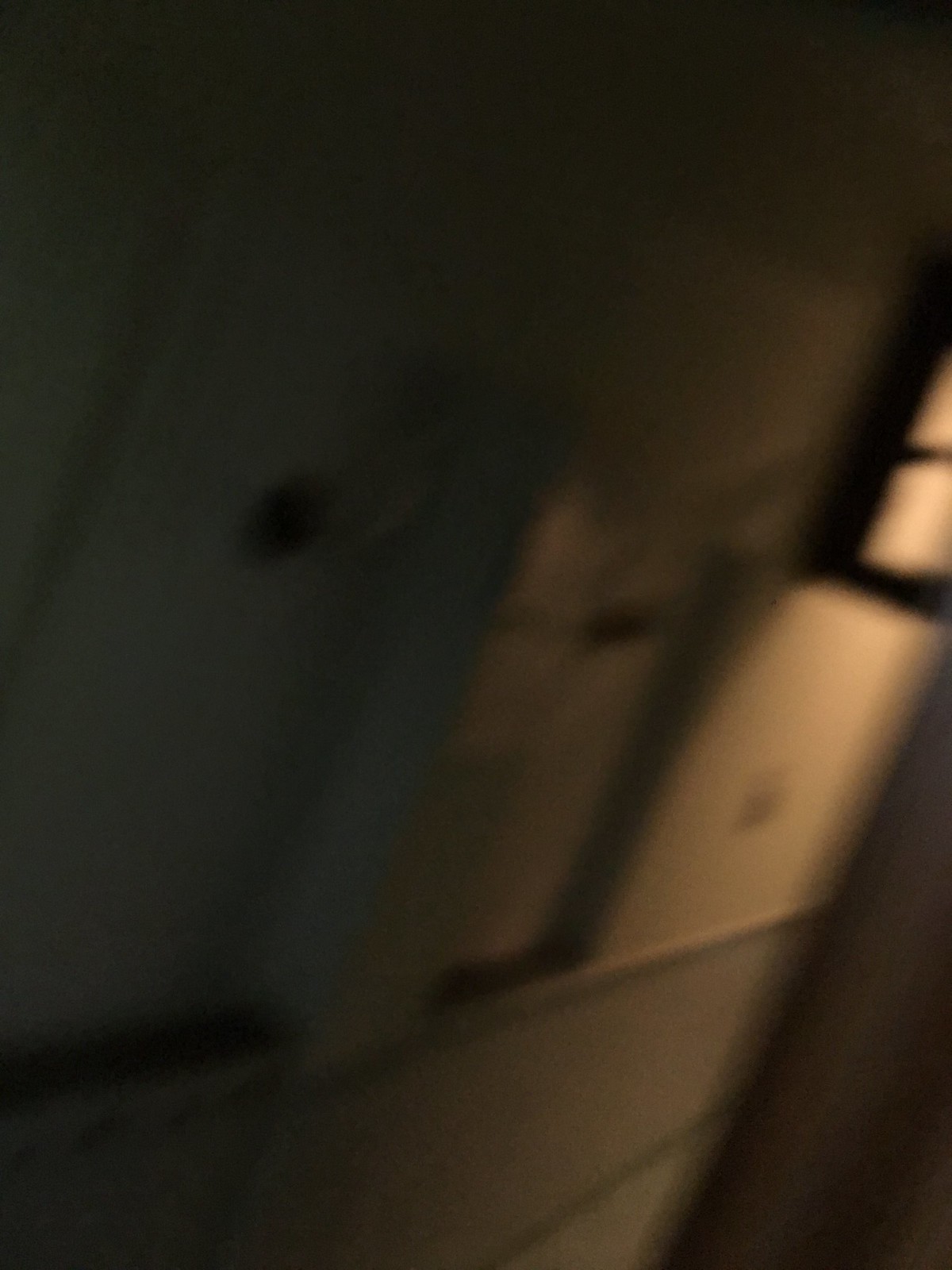A dimly lit and poorly focused photograph captures a mysterious and somewhat indistinguishable scene. The image, taken at an angle, shows a poorly illuminated wall with a slight slope upward to the right. The wall, rendered in a muted tan hue, features a somewhat visible light switch. Bathed in sparse light, the scene is enveloped in shadows, leaving much of the detail obscured. In the bottom right corner, a dark, indistinct object creates further obstruction, while a shadowy handle-like structure appears at the top, adding to the intrigue of the photograph. The overall ambiance is one of obscurity and uncertainty.